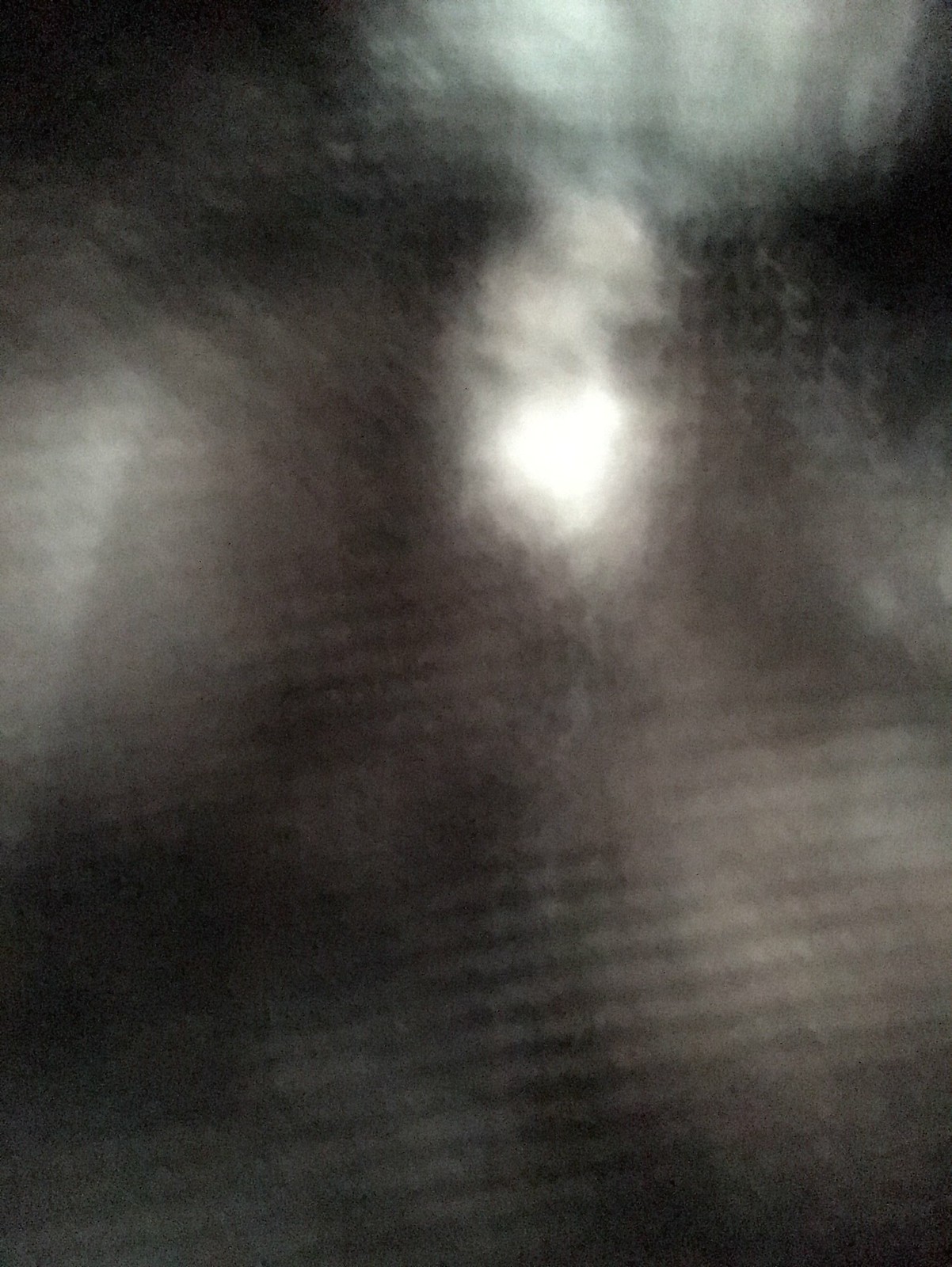The image depicts a night scene characterized by an incredibly blurry and indiscernible view, likely taken in low light conditions. The background is predominantly black, adding to the difficulty in distinguishing specific elements. In the upper right quadrant, there is a prominent circular object that appears gray and is bisected down the middle, occupying roughly 20% of the image's vertical span and 60% horizontally. Centered within the image are several tan-colored, circular shapes that vary in size. To the left, there's a significant circular form extending two-thirds inwards from the edge, while a similarly sized object is located in the lower right-hand corner. These are connected by a diffuse ball of light with a smoky trail above it. Across the scene, particularly in the top and bottom sections, there are areas of lighter gray and off-white hues interspersed with black spots and faint striations, resembling abstract outlines and forms, contributing to the eerie and indistinct nature of the photograph.